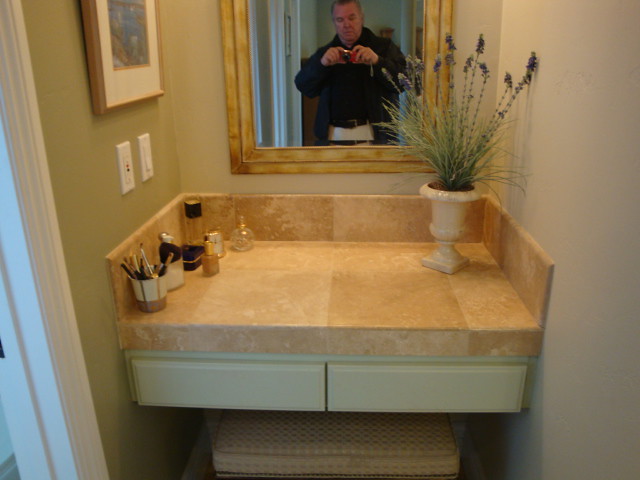In this photograph of a bathroom vanity, a large mirror above the vanity partially reflects the image of the photographer, a middle-aged man with gray hair, dressed in a black shirt, white pants, and potentially a jacket. The vanity countertop features brown marbled tiles and is adorned with various items. On the right and left sides of the countertop, there is an assortment of perfumes, beauty products, and makeup. A vase filled with what appears to be lavender is placed in the center of the vanity. Beneath the countertop, there are white drawers, and a stool is neatly tucked under the vanity. The walls of the bathroom are painted in a pale sage or beige color, and a white door frame is visible on the far left side of the photograph. Additionally, two electrical outlets are positioned on the left wall, above which a decorative picture is hanging.